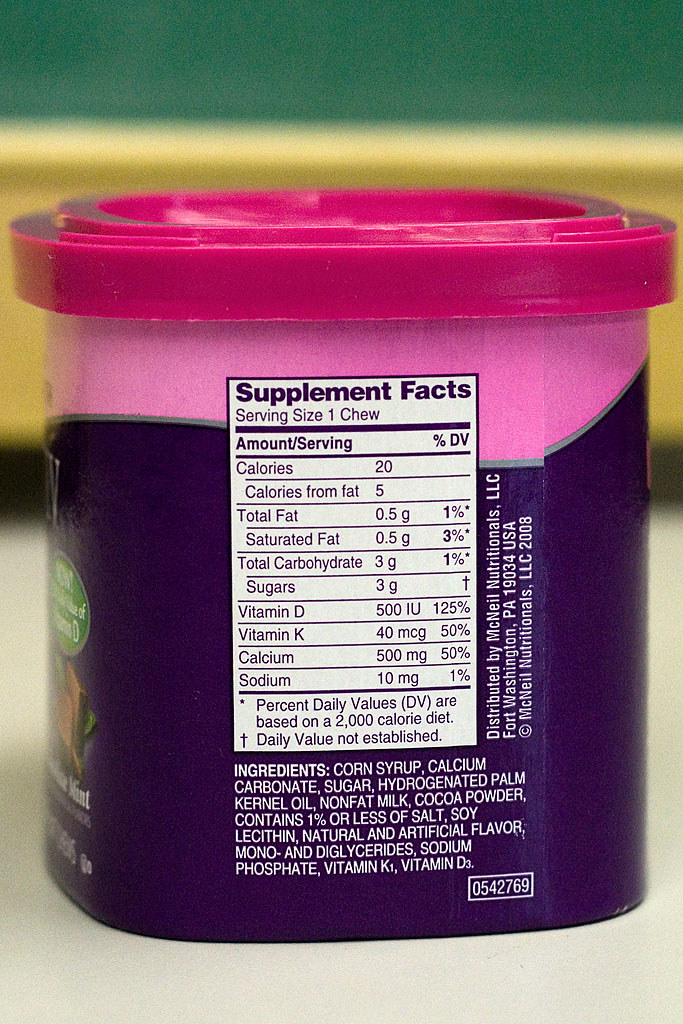This is a close-up photo of the side of a container, likely housing a type of nutritional chew supplement. The container is square-shaped with a bright fuchsia, snap-on plastic lid. The top portion of the container is pink, transitioning to a dark purple color at the bottom. The side of the container prominently displays the Supplement Facts, revealing a serving size of one chew, along with detailed nutritional information. Each chew provides 20 calories, with 5 calories from fat, 0.5 grams of total fat, 3 grams of total carbohydrates (all sugars), and small amounts of sodium (1%). The chew also supplies significant percentages of certain vitamins and minerals: 125% of Vitamin D (500 IU), 50% of Vitamin K (40 micrograms), and 50% of Calcium (500 milligrams). Below the nutritional information, a comprehensive list of ingredients starts with corn syrup, calcium carbonate, and sugar. Additionally, the container denotes the distributor's location in Pennsylvania and includes a copyright number.